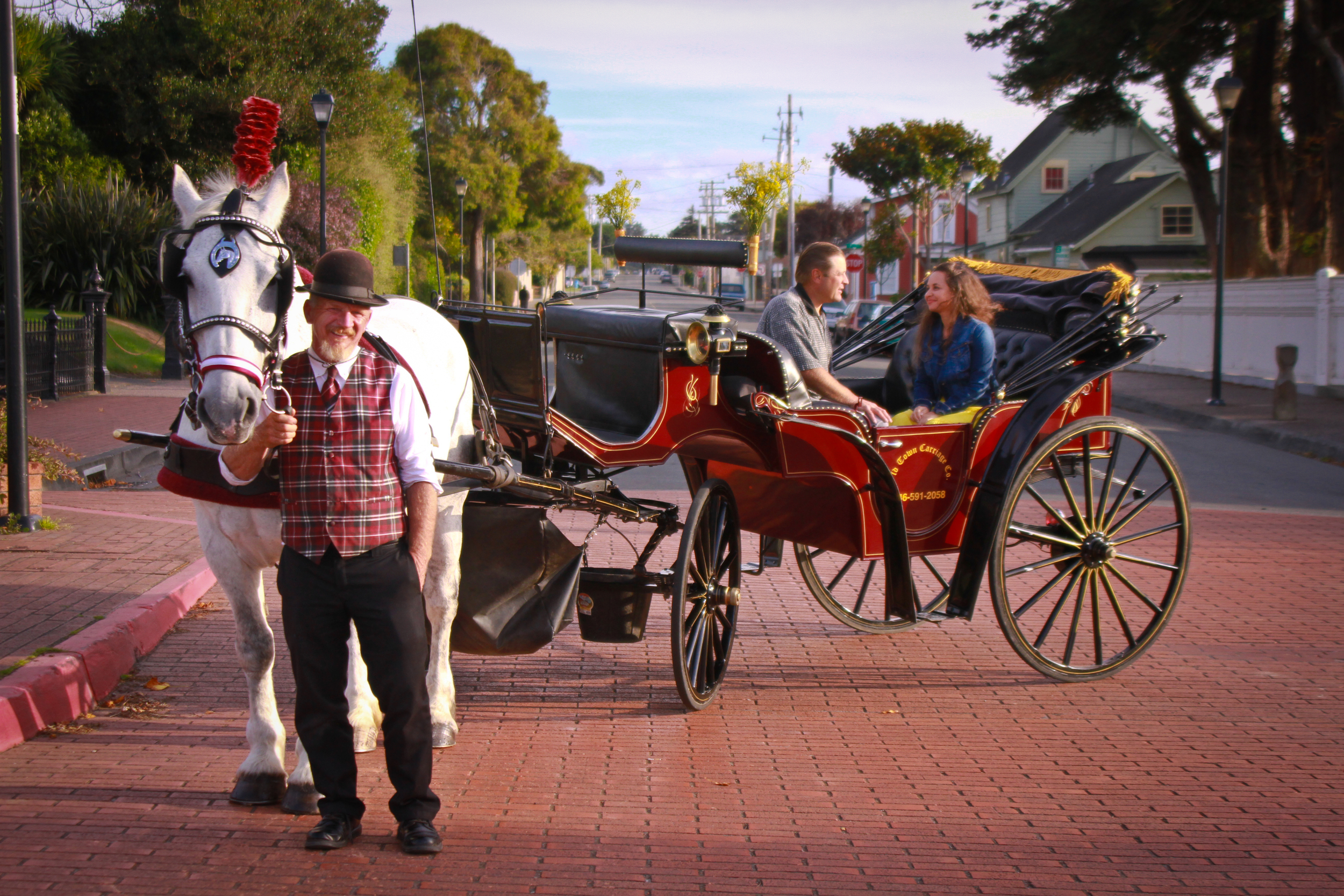In this vibrant street scene photograph, a charming red brick road stretches from the foreground to the center, flanked by a red painted curb and a matching red brick sidewalk on the left. Dominating the left side of the frame, a lamppost stands tall beside a white horse adorned with a red crest and a black bridle studded with silver dots. Next to the horse, a man with a white beard smiles warmly at the camera, dressed in black pants, shoes, and a plaid red vest over a white dress shirt with a red tie, topped off with a black bowler hat.

Attached to the horse is a striking red carriage featuring four gold-spoked wheels with black rims. On its door, the text "The Town Carriage Co." along with a phone number stands out in yellow. Seated in the open carriage, a man in a gray polo shirt with closely cropped brown hair and a woman in a denim jacket with a yellow skirt share a moment of connection. The carriage’s black convertible roof is down, allowing a clear view of the couple sitting against the black seat. 

The backdrop reveals a serene residential neighborhood, with a row of houses on the right and green trees lining a street that recedes into the distance, framing this picturesque and nostalgic tableau.